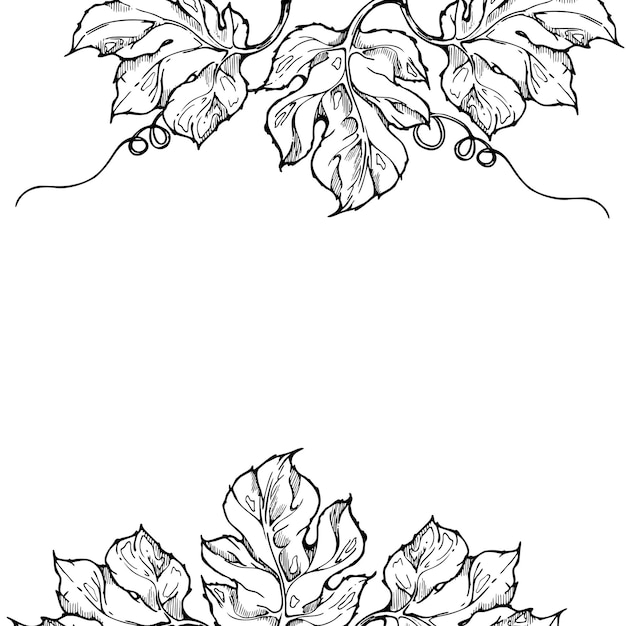This is a highly detailed, black and white pen drawing of grapevine leaves, featuring three leaves at the top and three at the bottom. The leaves, drawn with bold, thick black lines and accented with thinner lines for shading, each have five distinct "fingers" or lobes. The top trio of leaves is interspersed with elegant, twirling vines that are characteristic of grapevines, while the bottom trio does not have these spirals. The center of the image is an open, white space, creating a striking contrast with the elaborate detailing of the leaves. Some of the leaves exhibit small holes, adding to their textured appearance. The overall effect is reminiscent of classic, detailed botanical sketches, similar to the wallpaper patterns often seen in vintage settings.